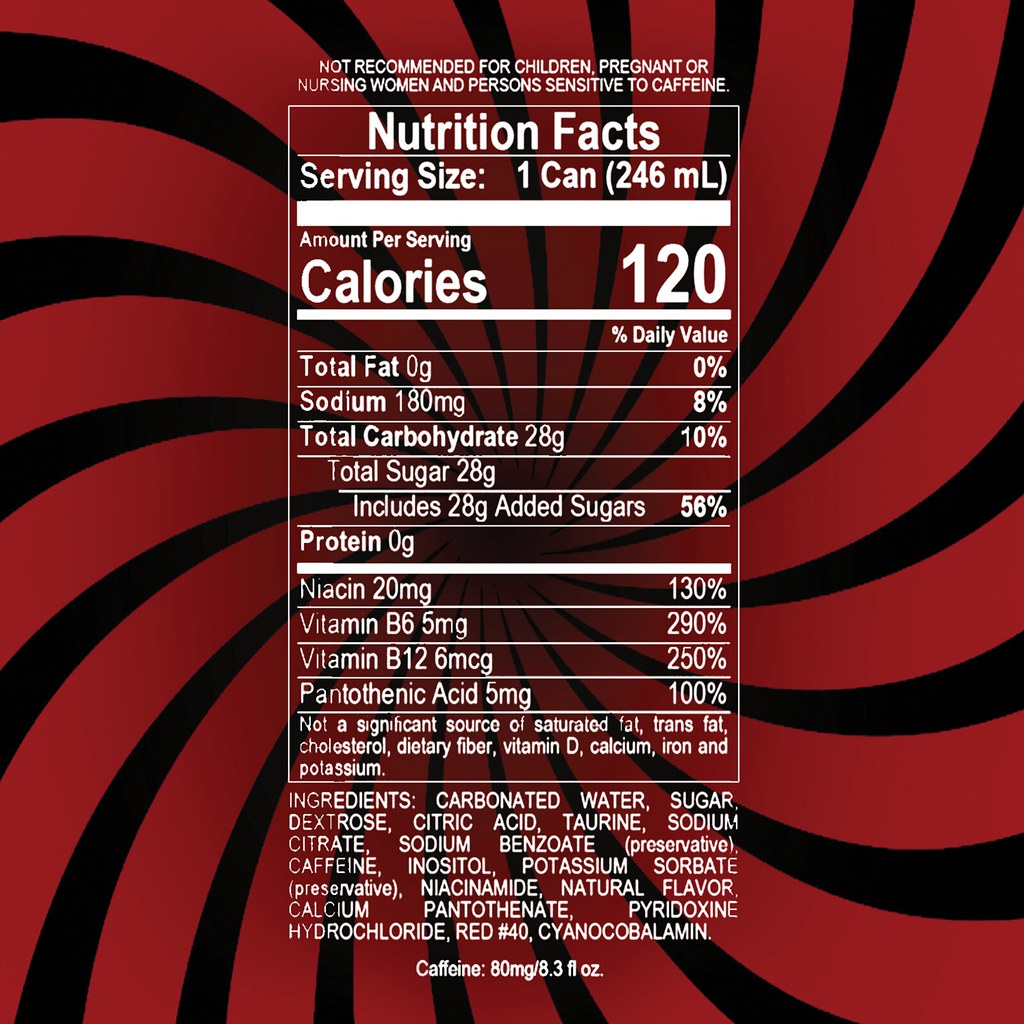The image showcases a nutrition label set against a striking black and red spiral background. At the top of the label, a cautionary statement reads: "Not recommended for children, pregnant or nursing women, and persons sensitive to caffeine." The label, appearing to be from a canned beverage, details that each serving size contains 120 calories. It highlights the following nutritional information: total carbohydrates at 28 grams and zero grams of protein.

The label systematically lists the following nutrition facts: calories, total fat, sodium, carbohydrates, and protein. It also provides specific amounts of various vitamins and minerals, including niacin, vitamin B6, vitamin B12, and pantothenic acid.

Beneath the nutritional facts, the label enumerates the ingredients, which include: carbonated water, sugar, dextrose, citric acid, taurine, sodium citrate, sodium benzoate (preservative), caffeine, inositol, potassium sorbate (preservative), niacinamide, natural flavor, calcium pantothenate, pyridoxine hydrochloride, Red #40, and cyanocobalamin. Additionally, it specifies that the product contains 80 milligrams of caffeine per 8.3 fluid ounces.